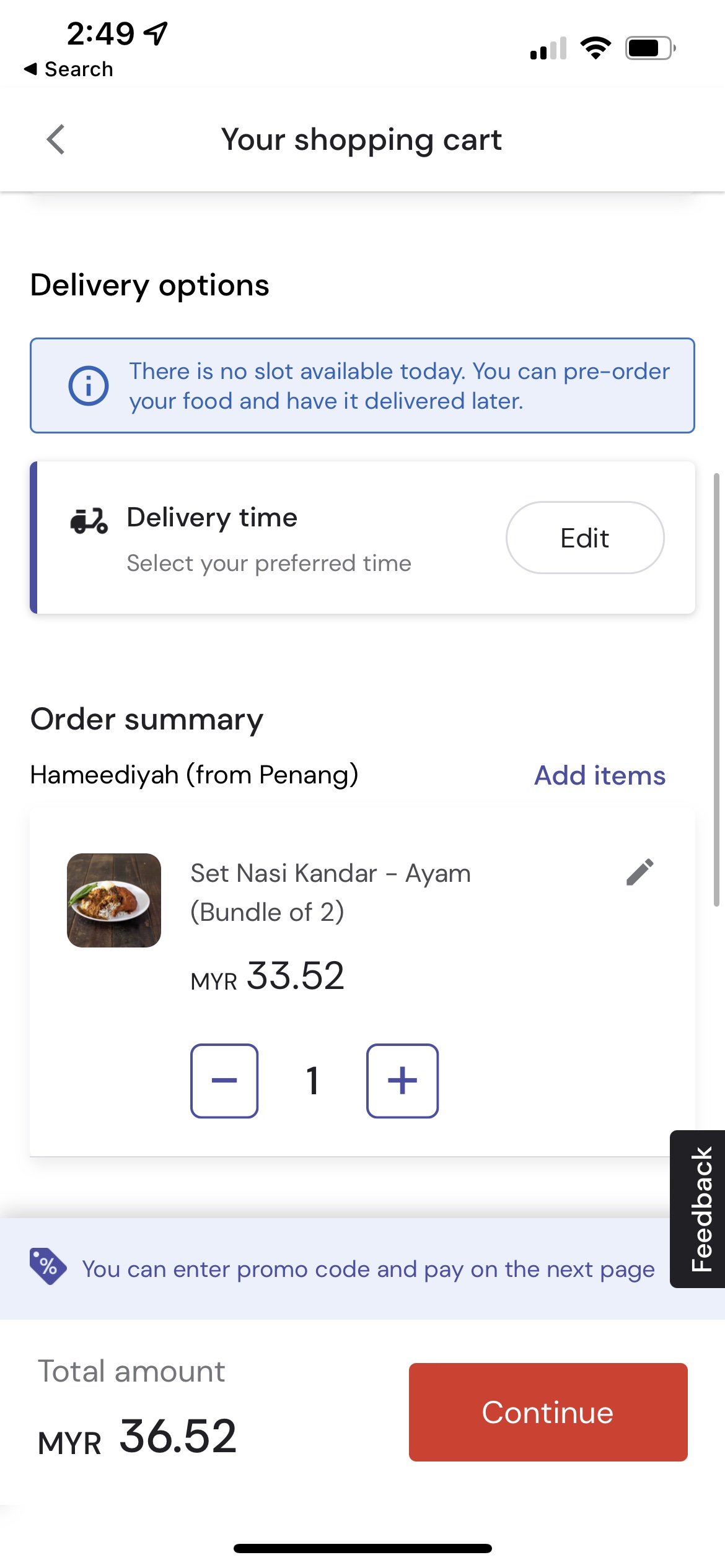The image depicts an online food delivery app interface. At the top of the screen, the time is displayed as 2:49 PM, alongside icons indicating full Wi-Fi signal, full battery life, and strong phone signal strength. Below these icons, a central shopping cart icon is visible, accompanied by a back button on the left side.

Centered on the screen is a section titled "Delivery Options," featuring a disclaimer in a light blue box that states, "No slot available today. You can pre-order your food and have it delivered later." Beneath this is a button labeled "Delivery Time," adorned with a truck image and a prompt to "Select your preferred time," with an edit button on the right side for changing the delivery time.

Following this, there is an "Order Summary" section. The summary indicates the order is from Penning, an Asian restaurant named Hameediah (H-A-M-E-E-D-I-Y-A-H). A button labeled "Add Items" on the right allows users to add more items to their order. Currently, the order consists of a bundle of two Nasi Kandar dishes. An adjacent pencil icon indicates the option to edit the order, such as changing toppings. There are also minus and plus buttons to adjust the quantity. 

Directly beneath the blue box for promo code entry, the total order cost displays as MYR 36.52. At the bottom of the screen, there is a red "Continue" button. Overlapping the promo code section is a sideways black button labeled "Feedback."